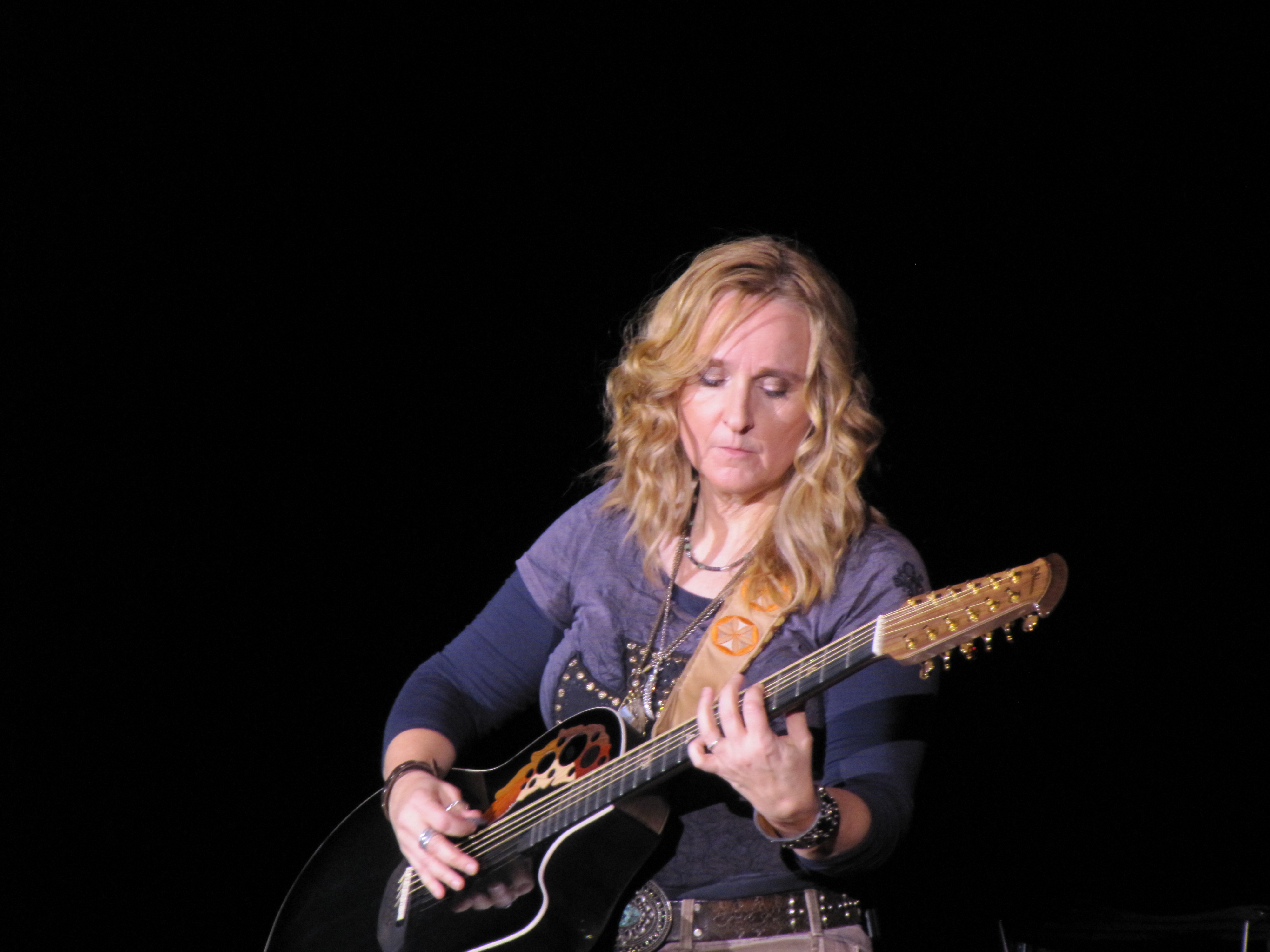The image captures musician-performer Melissa Etheridge during a concert, deeply engrossed in playing an acoustic guitar. Seated slightly to the right of the center, she's illuminated by a spotlight against a solid black background which accentuates her presence on stage. Etheridge's long blonde hair frames her face as she looks down intently at the instrument. She dons a long-sleeved shirt layered under an outer t-shirt, decorated with graphics and studded elements. A gold necklace hangs around her neck, and a notable belt with a large oval silver buckle cinches her outfit. The guitar, positioned with the headstock pointing to the right and the body angled down to the left, features prominently in the scene. The colors in the image range from light purple, blue, turquoise blue, red, orange, black, white, beige, and grays, adding a vivid and dynamic quality to the concert setting.